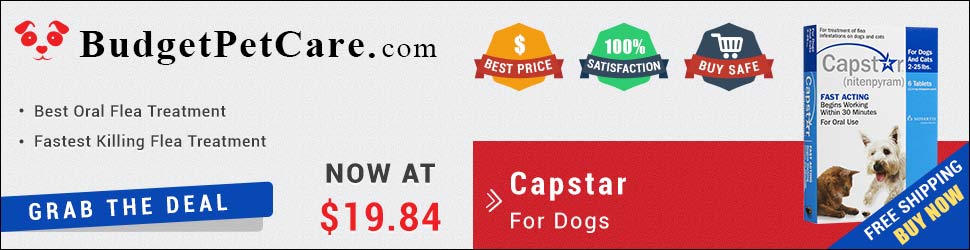This advertisement flyer for Budget Pet Care features multiple elements and detailed information about the showcased product, Capstar. 

On the left side, there is an image of a red dog, accompanied by the text "BudgetPetCare.com" in black. Adjacent to this, several icons highlight the benefits of the shop, including a "Best Price" icon, a "100% Satisfaction" icon, and a "Buy Safe" icon.

Central to the flyer is the featured product, Capstar. The packaging of Capstar is displayed prominently, showing a white and blue design. The product is described in detail with phrases such as "for dogs and cats, 2 to 25 pounds," "comes in tablets," "fast-acting," "begins working within 30 minutes," and "for oral use." Additionally, the flyer includes images of a brown cat and a white dog to signify the product's usability for both pets.

On the left side of the flyer, bold text emphasizes Capstar as the "Best Oral Flea Treatment" and the "Fastest Killing Flea Treatment." 

A prominent banner at the bottom of the flyer urges customers to "grab the deal now" at a price of $19.84. Additional promotional text mentions "Free Shipping" and prompts viewers to "Buy Now."